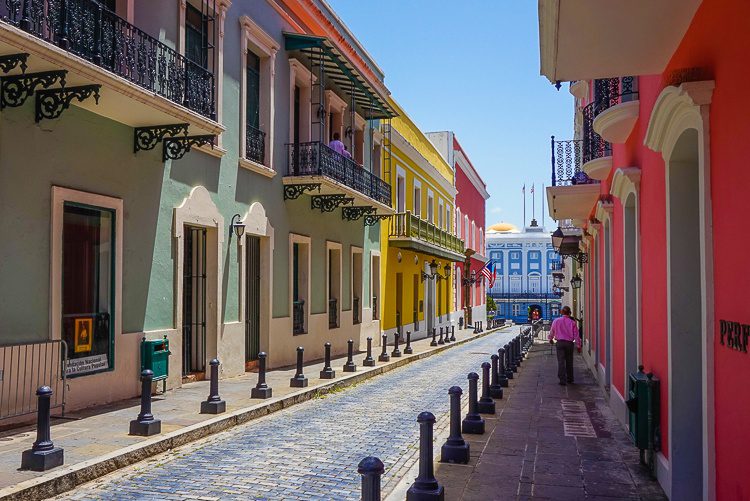This photo captures a vibrant street scene in a European city, potentially Denmark, Sweden, or even Amsterdam, marked by its distinct architectural features rarely seen in the United States. The street is paved with cobblestones and flanked by metal posts designed to keep cars within the roadway, ensuring pedestrian safety. The buildings lining the street are a lively mix of pastel colors, contributing to the picturesque ambiance. On the left side, the buildings progress from sage green to bright lemon yellow to red, each adorned with ornate, black balconies on their second levels. On the right, a bright pink building stands out, with arches marking its entrances and exits. A man dressed in a pink long-sleeved shirt and black pants walks along the right-side sidewalk toward the background. At the far end of the street, there's a striking building decorated in a blue and white delft China pattern, complete with three flagpoles atop its roof. The scene is set under a clear, blue sky, highlighting the vibrant colors and lively details of the street.